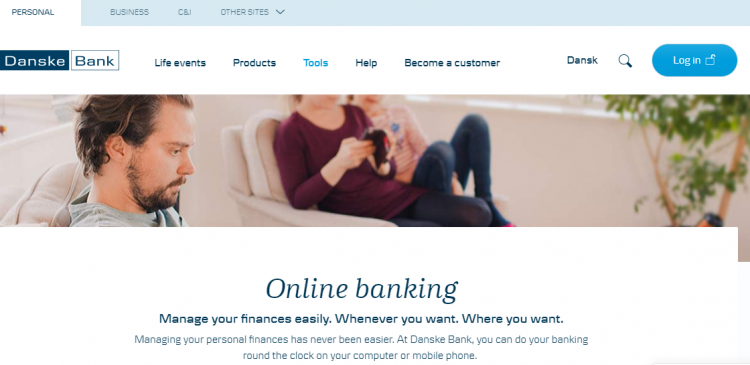The image depicts an online banking interface for Dansky Bank. The logo, "Dansky Bank," is prominently positioned in the upper left-hand corner, with "Dansky" enclosed in a green box and "Bank" in a white box. At the very top of the interface, there are navigation options labeled "Personal" and "Business," with the "Business" option highlighted in a light blue box. To the right, there is a drop-down menu that appears similar to those on C&J and other sites.

The visual features a man with brown hair, a beard, and a mustache, who is sitting in a chair and appears to be reading something. He is looking straight ahead. Next to him, in another chair, is a partial image of a woman and possibly her child, or two teenagers, wearing purple and pink shirts and jeans. Their heads are slightly cut off in the image. The woman is holding an item that is black with red on the outside. A plant is visible in front of them, and there is also a tree in the background.

Beneath this scene, a section titled "Online Banking" outlines the convenience of managing finances through Dansky Bank. The text promotes the ease of banking around the clock via a computer or mobile phone, suggesting that the depicted individuals might be engaged in online banking. The narrative emphasizes that managing personal finances has never been easier, aligning with the relaxed and focused demeanor of the subjects in the image.